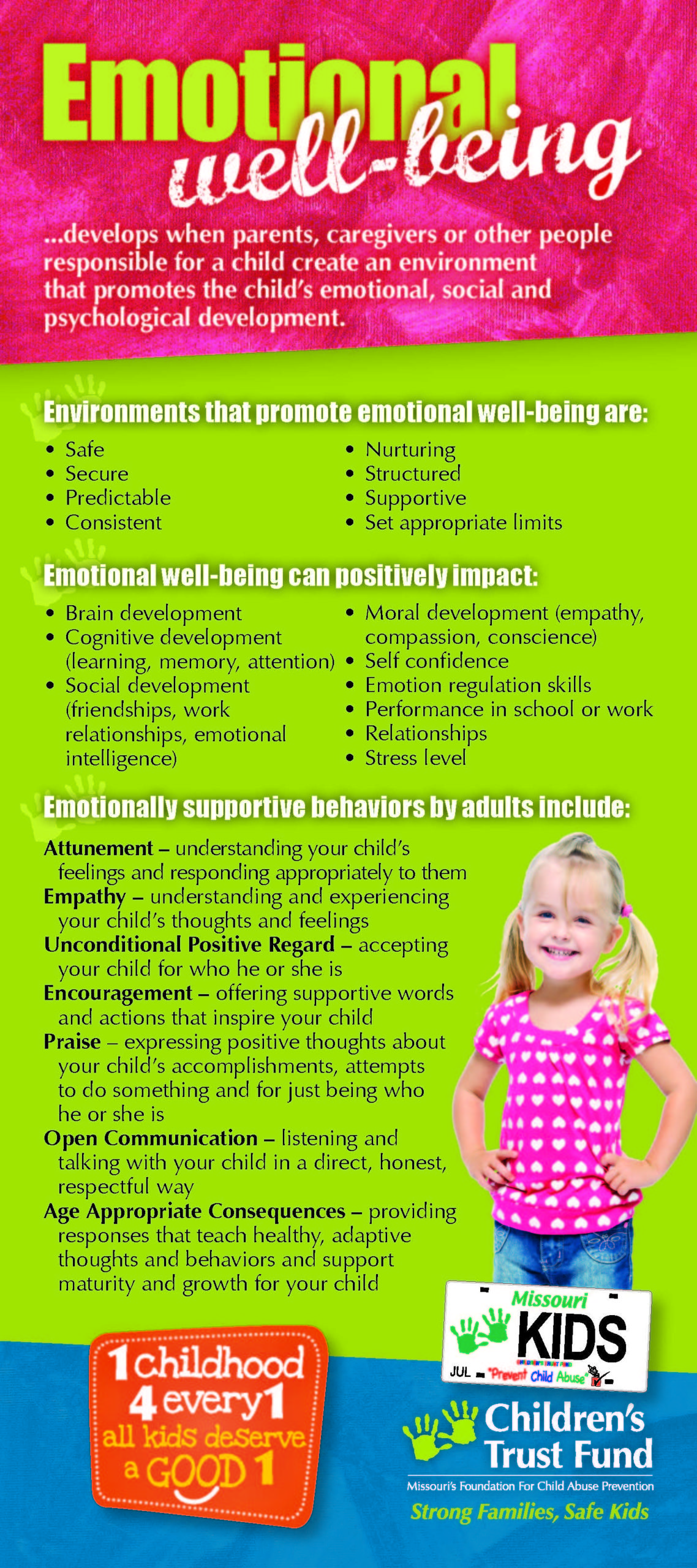The infographic, titled "Emotional Wellbeing," serves as a comprehensive guide to cultivating a supportive environment for children's emotional and social development. The title, prominently displayed in large yellow letters against a pink background, is followed by a defining statement in white letters: "Develops when parents, caregivers, and other people responsible for a child create an environment that promotes the child's emotional, social, and psychological development." The infographic is structured into three sections.

The first section, set against the pink background, introduces the topic. The main body, positioned against a bright lime green background, outlines various aspects of fostering emotional wellbeing. It details that environments promoting emotional well-being are characterized by safety, security, predictability, consistency, nurturing, structure, support, and appropriate limits. It further explains that emotional wellbeing positively impacts brain development and extends to relationships and school performance. Another detailed segment highlights supportive behaviors by adults, including attunement, empathy, unconditional positive regard, encouragement, praise, open communication, and age-appropriate consequences.

On the right side, an image of a young girl with blonde ponytails, dressed in a red and white polka dot blouse and blue jeans, adds a personal touch. Beneath her image, a Missouri license plate features the word "Kids" and two handprints, underscoring the involvement of the Children's Trust Fund. Below this, a blue background displays the organization's name in white letters with two handprints, and a red square on the left emphasizes the message: "One childhood for everyone. All kids deserve a good one," in white and yellow letters. This detailed layout aims to provide a clear and supportive framework for nurturing children's emotional and psychological health.